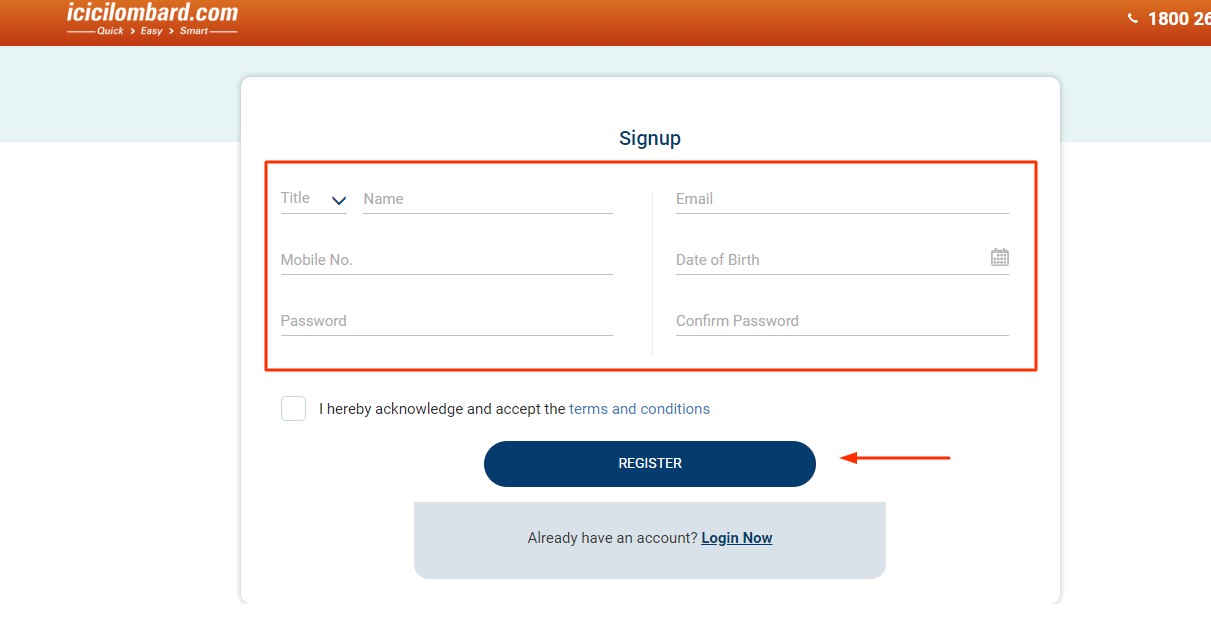Website Screenshot Description:

The webpage features an orange title bar at the top. On the upper left-hand side of the title bar, the website address is displayed as "ICICILombard.com" in clear, bold lettering. On the far right side of the bar, there is a partially visible toll-free phone number beginning with "1-800-26," though the rest of the number is cut off from view.

The body of the webpage starts with a gray background that extends about an inch from the top. The majority of the background below that is white. Prominently featured in the center of the page is a white pop-up box with black text prompting users to "Sign Up."

Inside the pop-up box, there are fields for user input within an orange-framed section. The fields include a drop-down menu for selecting a title, followed by spaces to enter a name, mobile number, password, email, date of birth with an adjacent calendar icon, and a field to confirm the password. 

Below these fields, there is a small checkbox next to the statement, "Hereby acknowledge and accept the terms and conditions." Underneath this statement is a button labeled "Register" for completing the sign-up process.